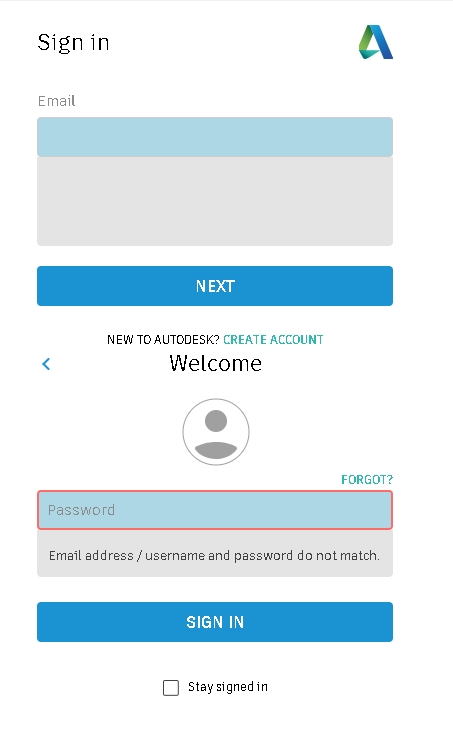This is a detailed and cleaned-up caption for the image:

---

The screenshot appears to be taken from a mobile device, such as a phone or tablet. The image prominently displays a user sign-in screen with a white background. 

In the top-left corner, the text "Sign in" is printed in black. On the top-right side, there is a stylized 'A' logo in blue and green.

Below this, on the left side, the word "Email" is visible, alongside a gray input box with a light blue bar at the top, which is currently empty. Directly underneath, there is a long blue button that reads "Next."

Following the button, the text "New to Autodesk?" appears, inviting users to create a new account. This text is accompanied by a blue link that says "Create account." Beneath this, the word "Welcome" is displayed, followed by a left-pointing caret symbol and an icon representing a person. The icon consists of a circle for the head and an elongated oval for the torso.

To the right of the person icon, the text "Forgot?" in blue is visible, indicating a forgotten password link. The password input box below it is highlighted in red, signaling an error.

Beneath the password box, a message in a gray box reads, "Email address/username and password do not match." Below this error message, there is a dark blue button labeled "Sign in."

At the bottom of the screen, there is a check box next to the text "Stay signed in."

---

This caption furnishes a clear and detailed description of the elements present in the screenshot.